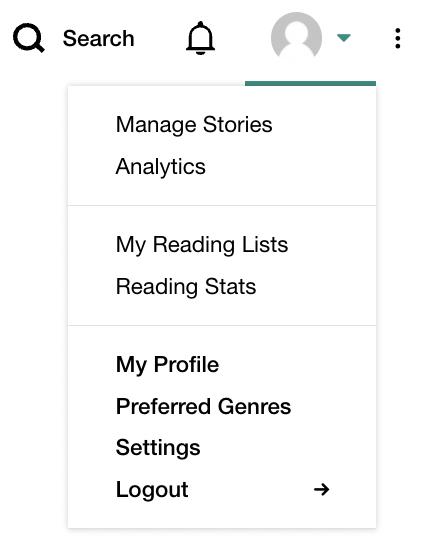The image starts at the top of the page, set against a clean white background. In the upper left corner, there is a bold black magnifying glass icon with a white center. Next to it, in bold black font, the word "Search" is displayed. Following this, there is a black bell icon, and to its right, a gray circle featuring a white silhouette of a person.

Below the silhouette, there is a green triangle pointing downwards, with a bold green underline extending underneath both the silhouette and the triangle. At the far right edge of this section, there are three vertical dots aligned in a column.

In the center of the page, there is a vertically oriented rectangular image divided into three sections. The first section contains the text "Manage Stories" and "Analytics," both in black font. A faint line separates this section from the next. The second section reads "My Reading Lists" and "Reading Stats," again with each word capitalized at the beginning. Another faint line separates these words from the final section.

The last section, written in bold black font, includes "My Profile," "Preferred Genres," "Settings," and "Logout." To the right of "Logout," there is a bold black arrow pointing to the right.